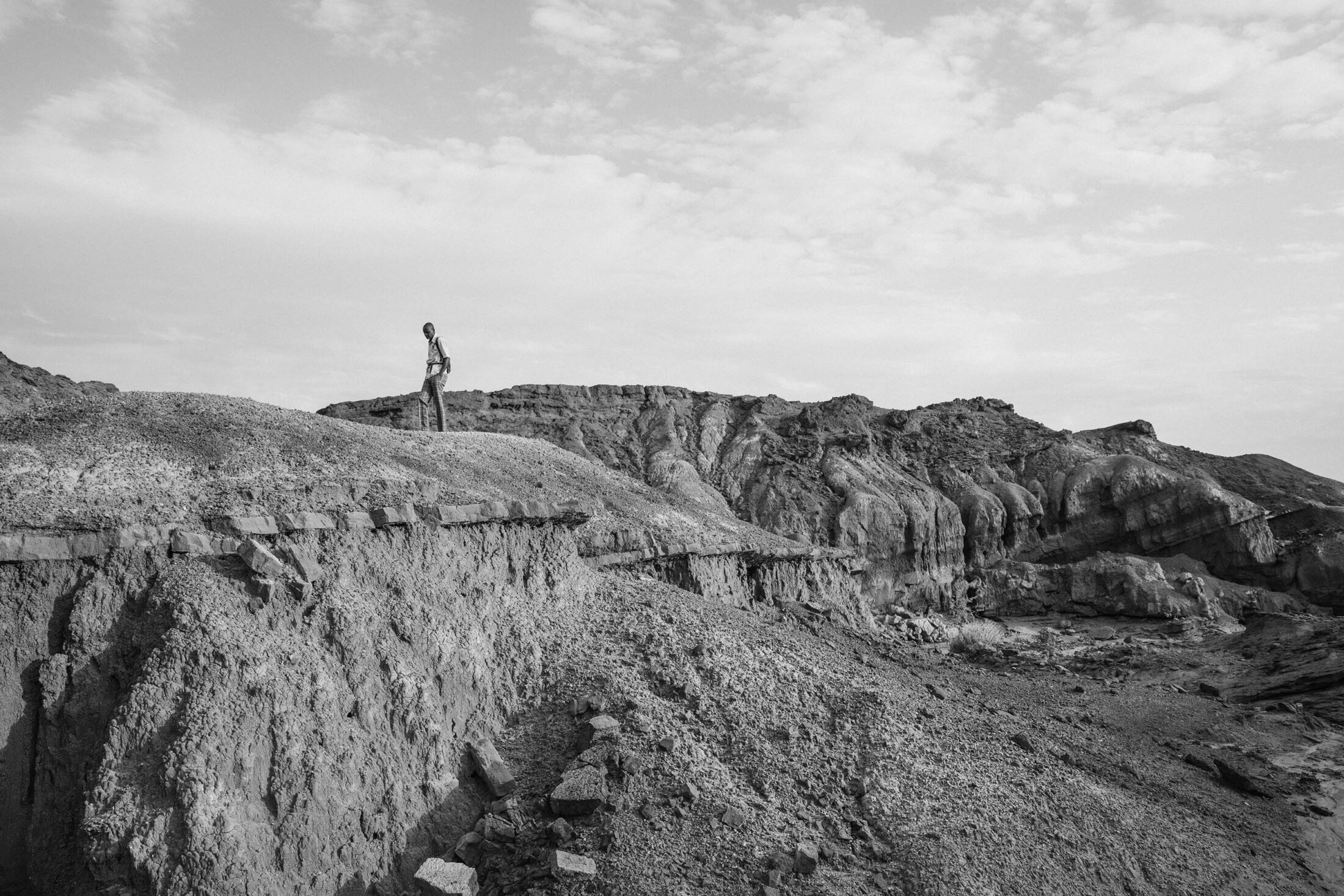In this detailed black and white photograph, a young Black man stands on a rugged, rocky hillside, possibly part of an expansive and arid landscape similar to the Grand Canyon but not definitively so. The terrain, devoid of any vegetation, showcases sharp, jagged edges and layers of striated rock formations, suggesting significant geological history. Gravel and small chunks of stone scattered across the ground enhance the raw, rustic feel of the environment. The man, dressed in shorts and a shirt, is positioned off-center to the left, gazing downwards, adding a sense of solitude to the scene. Above him, a sky filled with white clouds suggests a sunny day, casting shadows on the terrain and highlighting larger fallen rocks in the foreground. In the background, faint walking paths cut through the dry, rocky valley, hinting at the natural pathways worn over time in this desolate yet striking landscape.